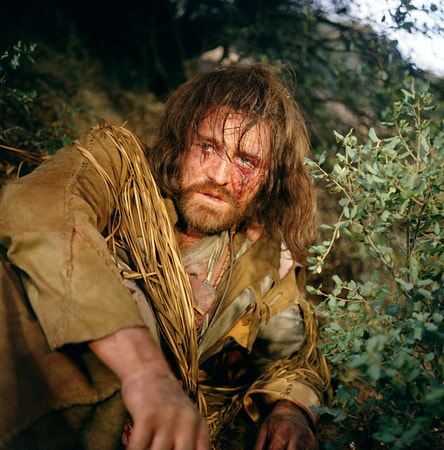In the center of a dense forest, a wounded man is seen either sitting or heavily lying on the ground, exhibiting an air of desperation. He has long, brown, disheveled hair that reaches his shoulders, and his rugged face, partially obscured by his hair, bears a fresh wound underneath his left eye. Sporting a brown beard and mustache, his appearance is that of a worn-out frontiersman, akin to historical figures like Davy Crockett or Daniel Boone. His attire consists of a shredded leather jacket and a distinctive scarf or poncho tied in front, seemingly made of straw and draped over his shoulders in tattered strips. His grayish-brown outfit is dirtied from the wilderness, complemented by his dirt-encrusted hands. The setting around him includes green plants to the right and a backdrop filled with more greenery, with a portion of the sky visible in the top right corner, enhancing the sense of isolation and turmoil within the image.